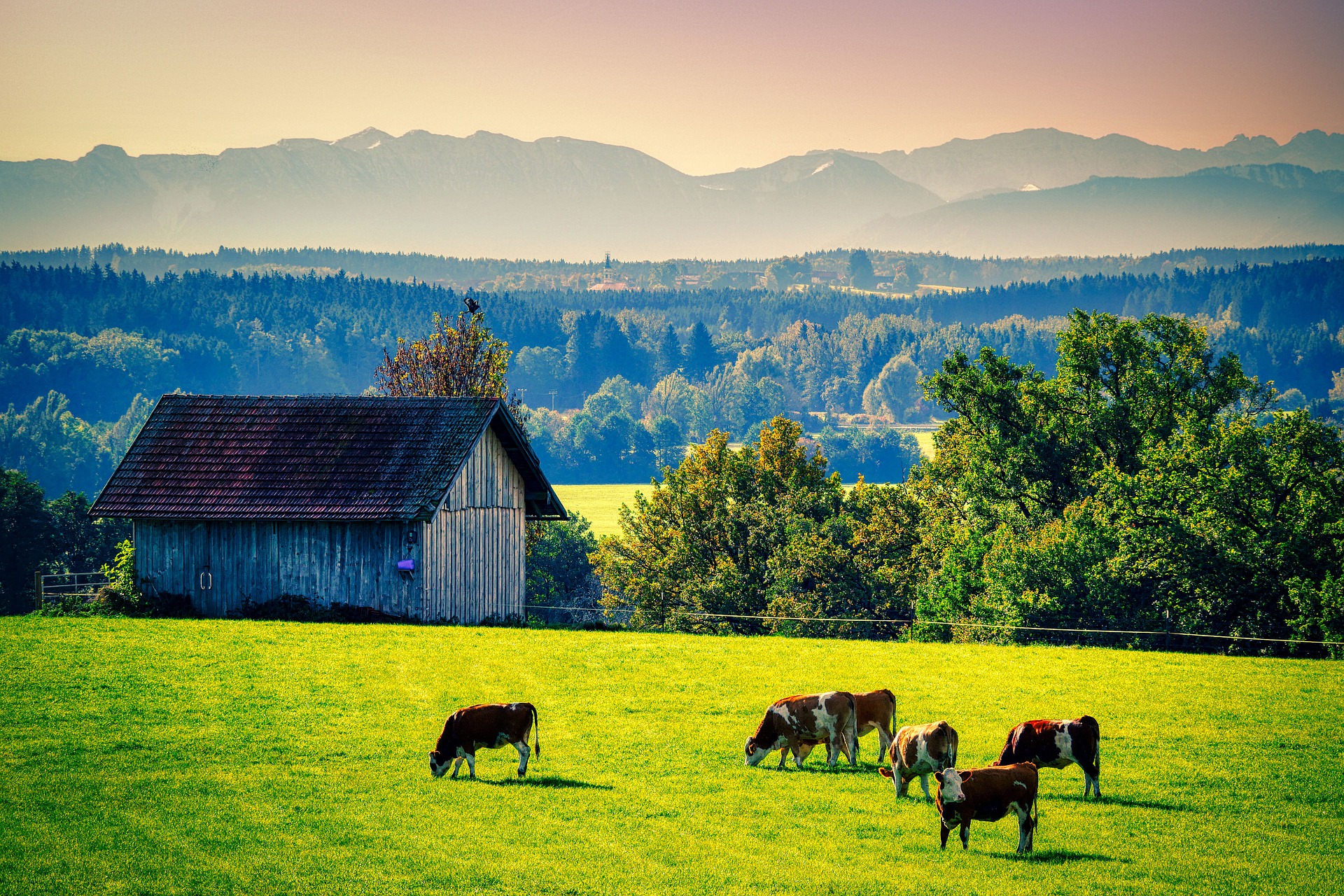This photograph captures a serene pastoral scene brimming with details. In the foreground, a bright green field occupies the bottom quarter of the image, where six cows, predominantly brown with some sporting white spots, graze. Notably, a brown cow with a white face in the bottom right corner gazes to the right, adding a touch of curiosity to the scene. To the left of the field stands a gray wooden barn with distinctive purplish shingles on its sloped roof. Adjacent to the barn, a copse of lush green trees adds density to the landscape. Beyond this, another expanse of green fields stretches out, leading to a sloping forested hill comprised of various yellowish and green trees. Rising above the treetops, a church steeple with a pointed green top punctuates the serene setting. Further in the background, a silhouetted line of mountains frames the horizon, above which an orange and pink gradient sky occupies the top fifth of the frame, suggesting the photo was taken during a striking sunset. This wide-angle view beautifully encompasses the tranquil farm and the extensive natural landscape that surrounds it.